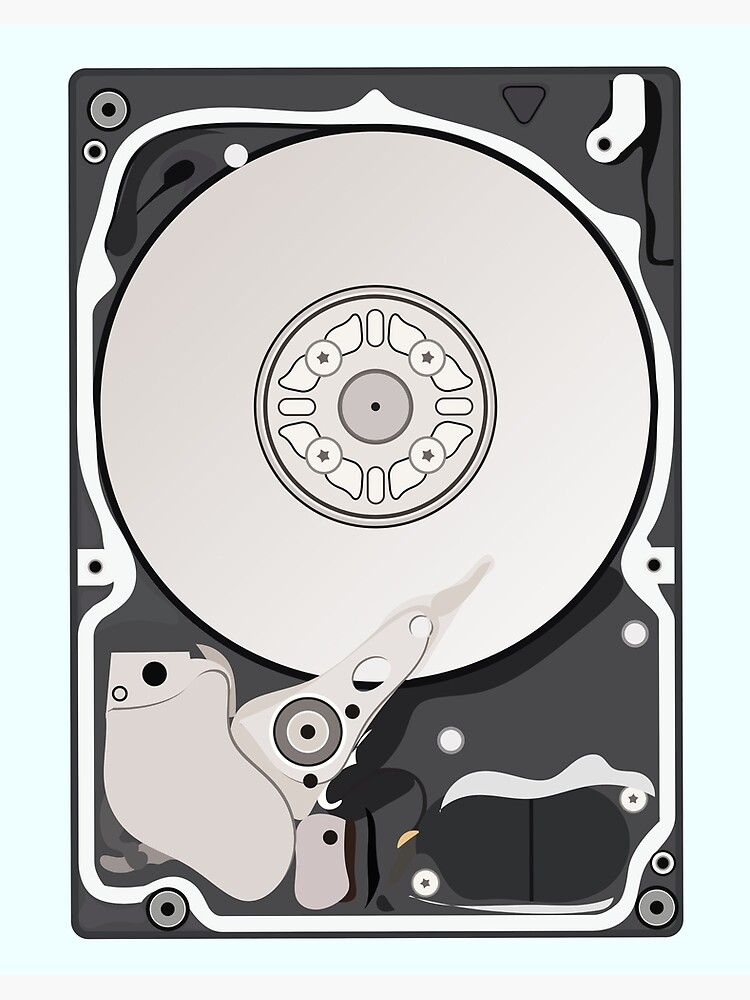The image is a detailed digital photograph of the underside of a modern-day hard drive. The central feature is a large, round, silver disk mounted in the center of the device. Surrounding this disk is a dark gray background, creating a striking contrast. At the bottom left corner of the image, you can see the hard drive's moving parts, featuring silver components including a prominent blade-like structure. The hard drive itself is primarily black, but various elements within it show silver and gray hues, with hints of light green and bronze. Multiple screws are visible, contributing to the intricate assembly of the device. The order of the objects gives a sense of cloud-like layers, enhancing the complex yet organized appearance of the hardware.